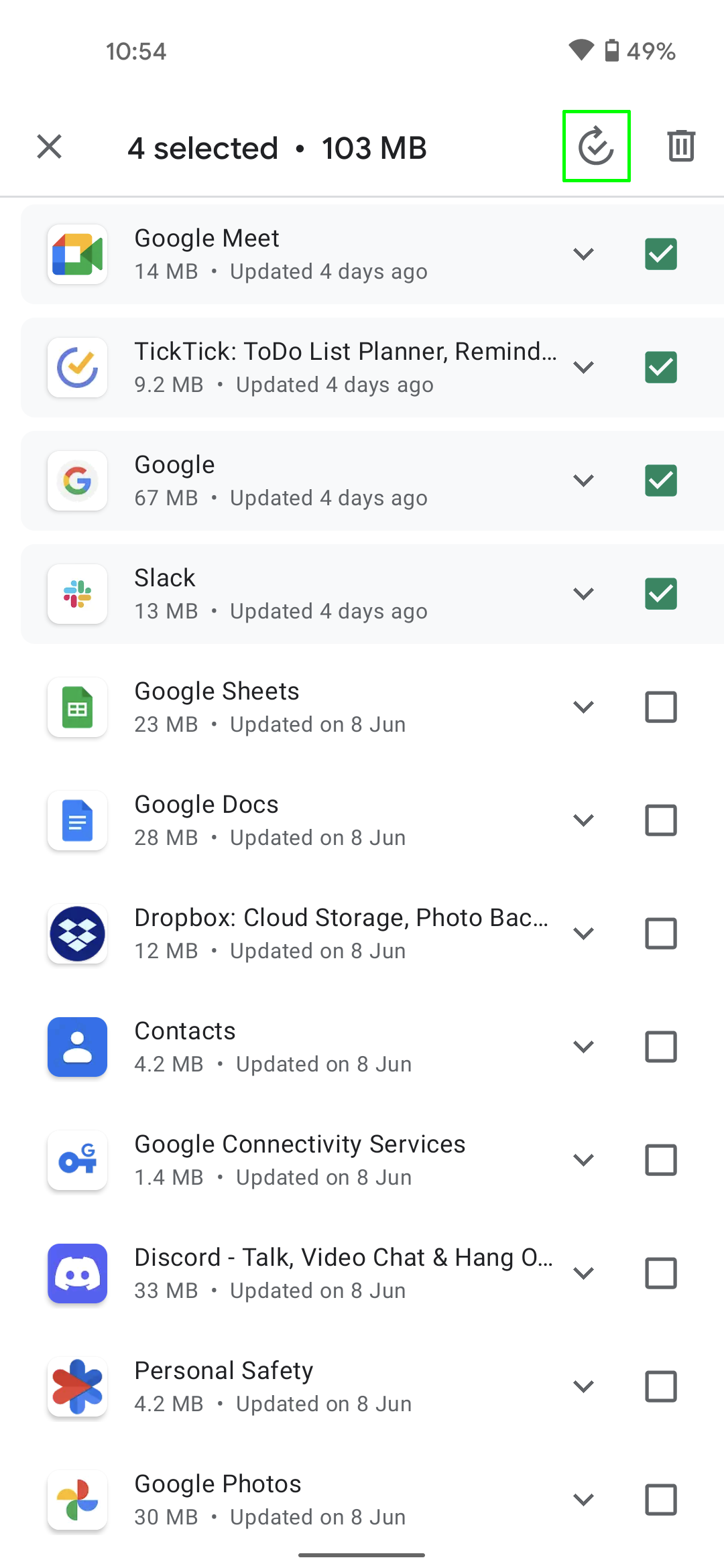In the screenshot displayed, the top left corner indicates the device time as 10:54. On the top right, the Wi-Fi icon and the battery icon are visible, with the battery level at 49%. The main content of the screenshot shows a Play Store page where various apps can be selected. The selected apps are Google Meet, TikTok, Google, and Slack. Additionally, a range of other apps is listed, including Google Sheets, Google Docs, Dropbox, Cloud Storage, Photo Backup, Contacts, Google Connectivity Services, Discord, Talk, Video Chat, Hangouts, Personal Safety, and Google Photos, none of which are selected. At the bottom of the image, the Navigation Pill button is visible.